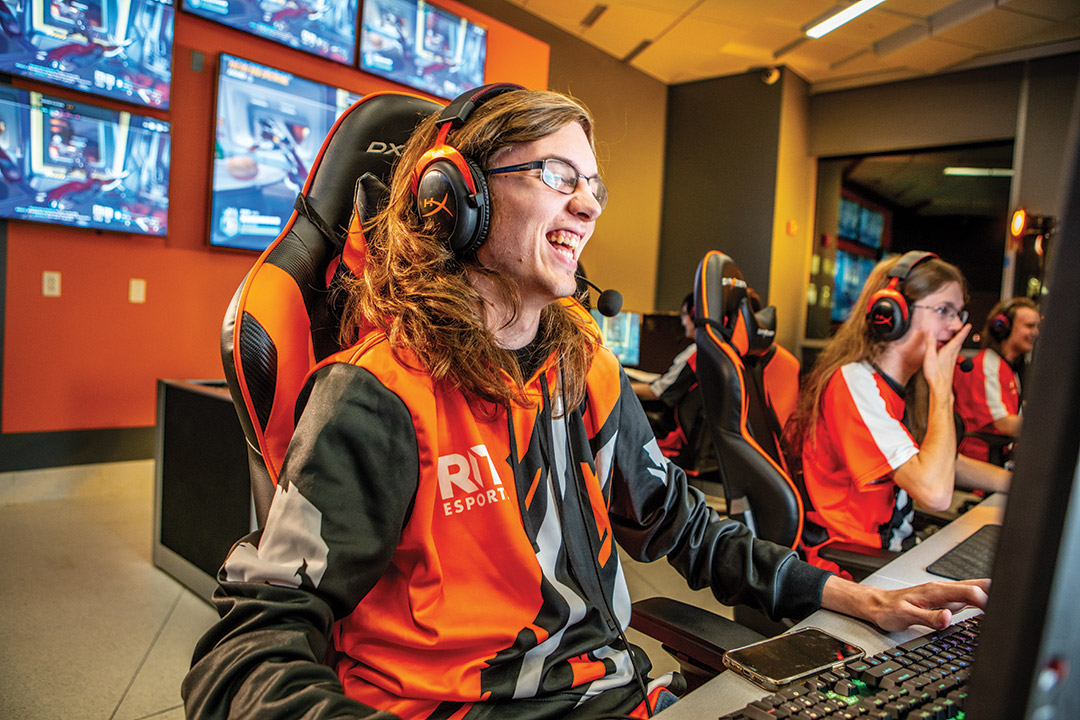The image captures a vibrant eSports competition scene featuring a group of gamers engrossed in their games. The focal point is three gamers seated at a table with numerous computer monitors and keyboards. All three are equipped with orange-accented black headphones and are seated in matching dark gray and orange gaming chairs. The gamer in the forefront, who appears to be mid-laugh or mid-smile, has long hair and wears black-framed glasses. This individual sports an orange jacket with black sleeves emblazoned with “RIT eSports.” Another person with long hair and similar headphones sits beside them, partially off-screen. Behind these gamers, the background is characterized by a vivid orange wall adorned with TV monitors displaying in-game footage, though the content is not clearly visible. The ambient light from the computer screens creates a bright foreground contrast against the slightly out-of-focus background. The room buzzes with concentration and energy, capturing the essence of an intense eSports competition.